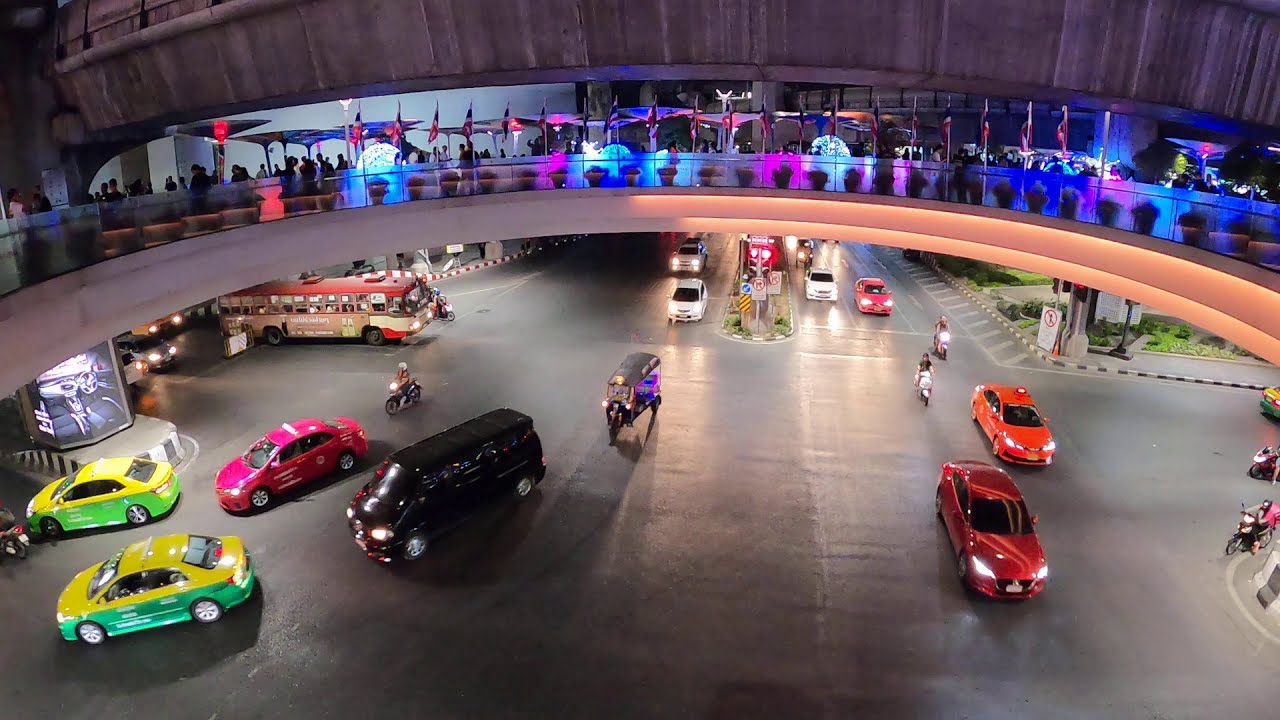The photograph captures a vibrant cityscape at a large, bustling intersection beneath a circular, arched balcony or bridge structure. The balcony, made of concrete, is adorned with numerous lights in hues of red, blue, and purple, creating an illuminated atmosphere. Approximately twenty flagpoles stand prominently towards the middle of the balcony. Below, the intersection comprises four to six lanes leading in multiple directions, filled with diverse vehicular traffic, including two green cars, a red car, a black SUV, and a distinctive red and white bus. Motorcyclists wait at the junction, adding to the lively scene. This setting, evocative of a bustling metropolis like Tokyo, also shows many people mingling on the balcony, enhancing the sense of urban vibrancy.